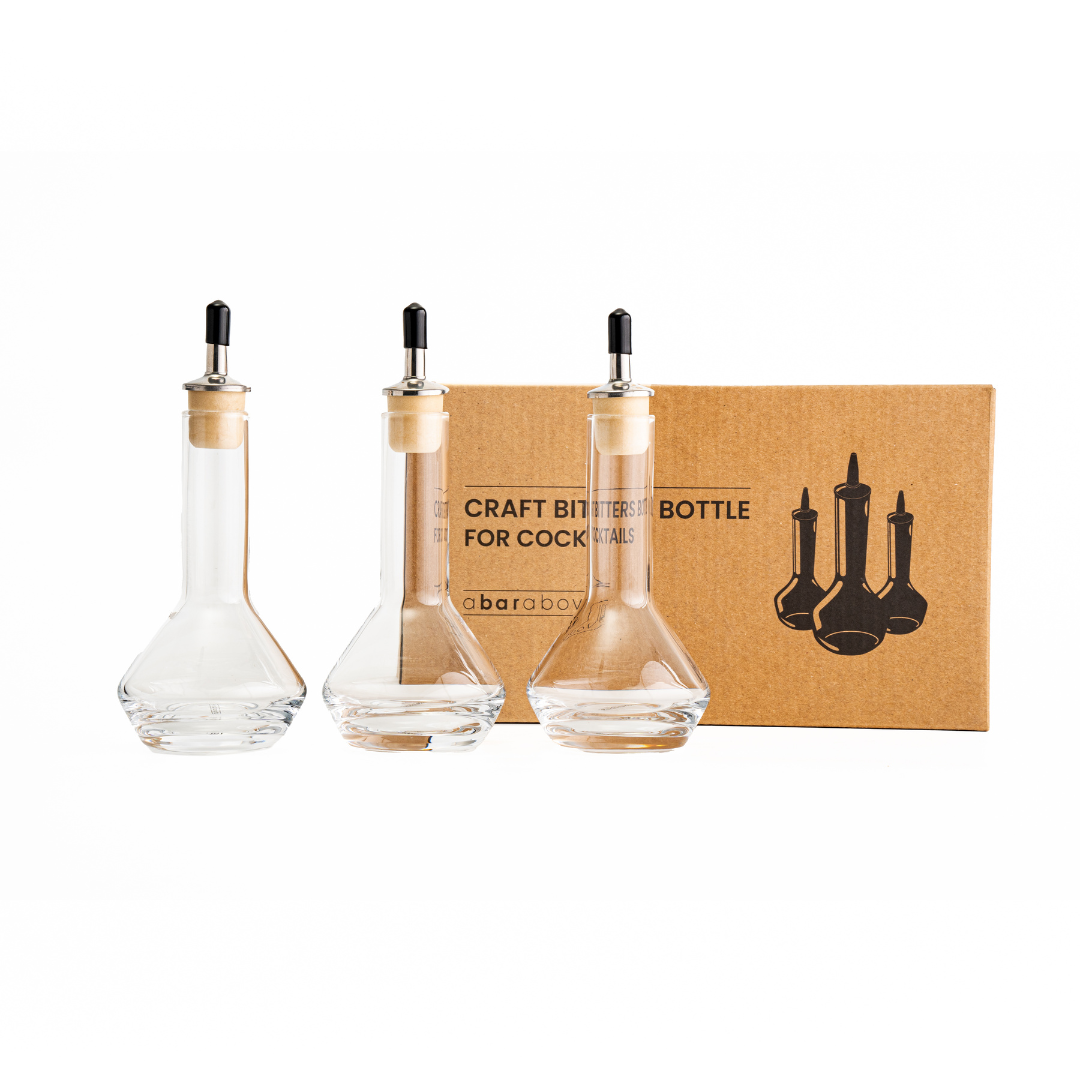The photograph displays three clear glass bottles, each resembling beakers with a thick base that tapers upward to a narrow opening. These bottles are fitted with cork stoppers, which are attached to metallic handles. The three bottles are aligned side-by-side in front of a brown cardboard box. This box, shorter than the bottles, features a drawn image of the three bottles and is labeled "Craft Bitters Bottle for Cocktails" along with the phrase "A Bar Above." The background of the image is plain white, highlighting the details of the bottles and the packaging.